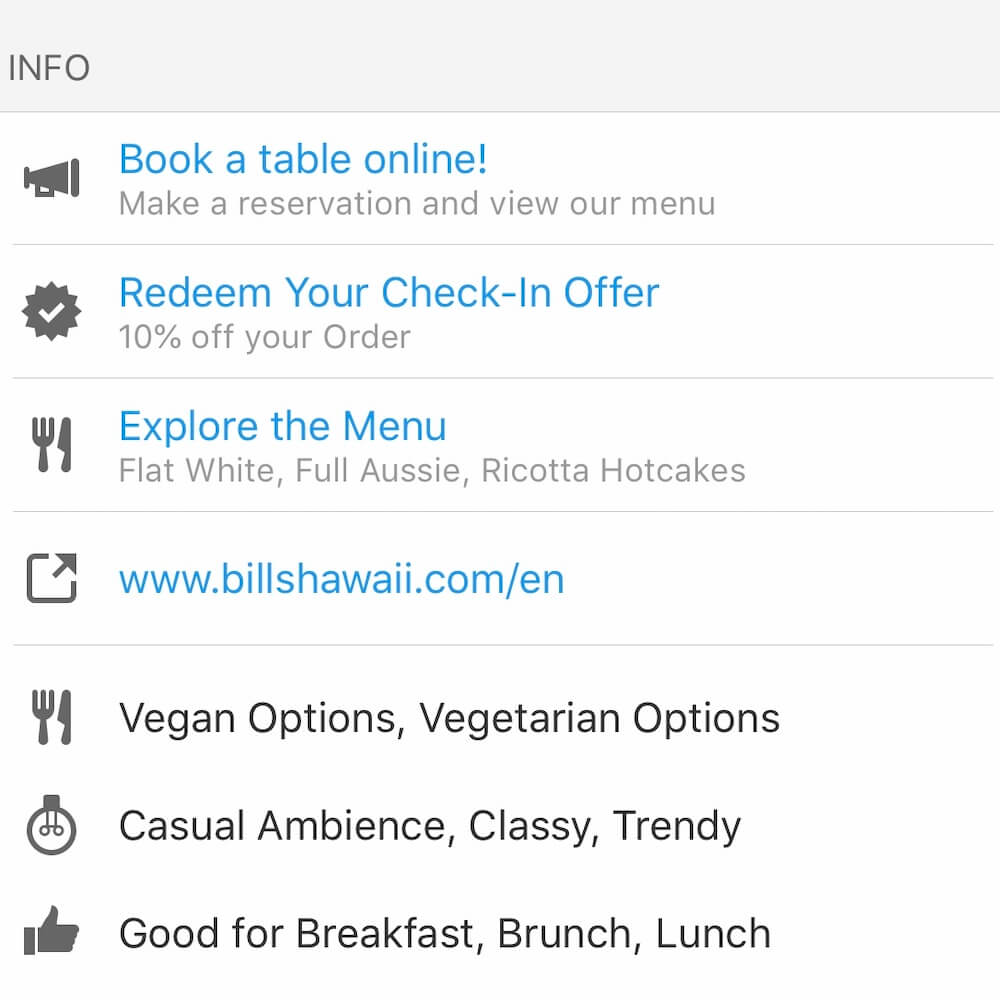Here's a detailed and cleaned-up caption:

---

A detailed view of a restaurant's website interface, presented in a near-square, portrait orientation. The background is predominantly white, complemented by a pale gray bar at the top. On the left side, there is a vertical, all-caps label reading "INFO." The white space of the screen is sectioned into various rows by thin gray lines, each row providing specific information.

The top row features a small gray megaphone icon, followed by the text "Book a table online!" in blue, with an exclamation point. Beneath this, in gray, it reads "Make a reservation and view our menu."

The second row highlights a pointed outline circle seal with a checkmark icon. Next to it, in blue, it says "Redeem your check-in offer," with the subtext in gray stating "10% off your order."

In the third row, there's a fork and knife icon. The accompanying blue text says "Explore the menu," and beneath it in gray, it lists menu items: "Flat White, Full Aussie, Ricotta Hotcakes."

The fourth row contains a blue hyperlink: "www.buildshawaii.com/EN."

The next three rows are unique: they are gray and do not have dividing lines between them. They contain gray icons and text describing various features. The first row mentions "Vegan options, Vegetarian options." The following row lists "Casual ambiance, Classy, Trendy." The final row describes the suitable dining occasions as "Good for breakfast, brunch, lunch."

---

This caption provides a detailed description of the visual elements and the information conveyed by each section of the restaurant's website.